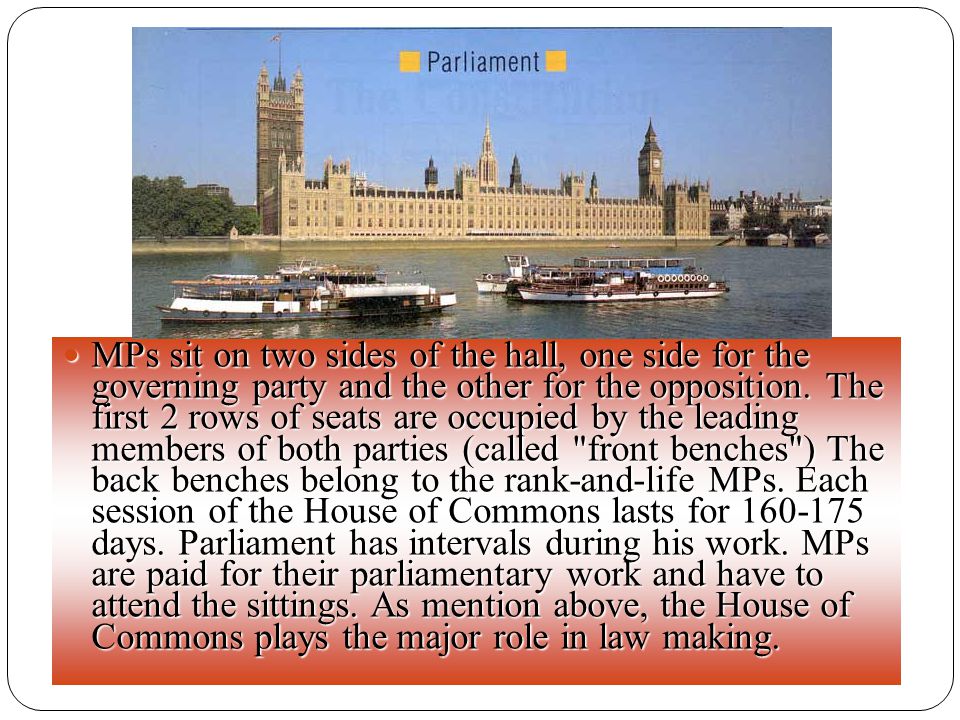The image depicts a large, long building identified as the Parliament, situated at the top with a river in front of it. In the foreground on the river, there are three boats, with two visible on the left and one on the right. The scene includes some flags, and the entire image is framed in a rectangular box with rounded corners and outlined in blue. The background is white, and the setting appears to be a daytime, outdoor scene. Below the image, there is a prominent red rectangle containing black text that describes the workings of the Parliament. The text explains that MPs sit on two sides of the hall, with one side for the governing party and the other for the opposition. Leading members of both parties sit in the first two rows called front benches, while the back benches are for the rank-and-file MPs. It also notes that each session of the House of Commons lasts between 160 to 175 days, with intervals in between. MPs are salaried for their parliamentary work and are required to attend sittings, and the House of Commons plays a major role in lawmaking. The colors present in the image include blue, yellow, brown, green, red, pink, and black, contributing to the detailed and informative presentation format.